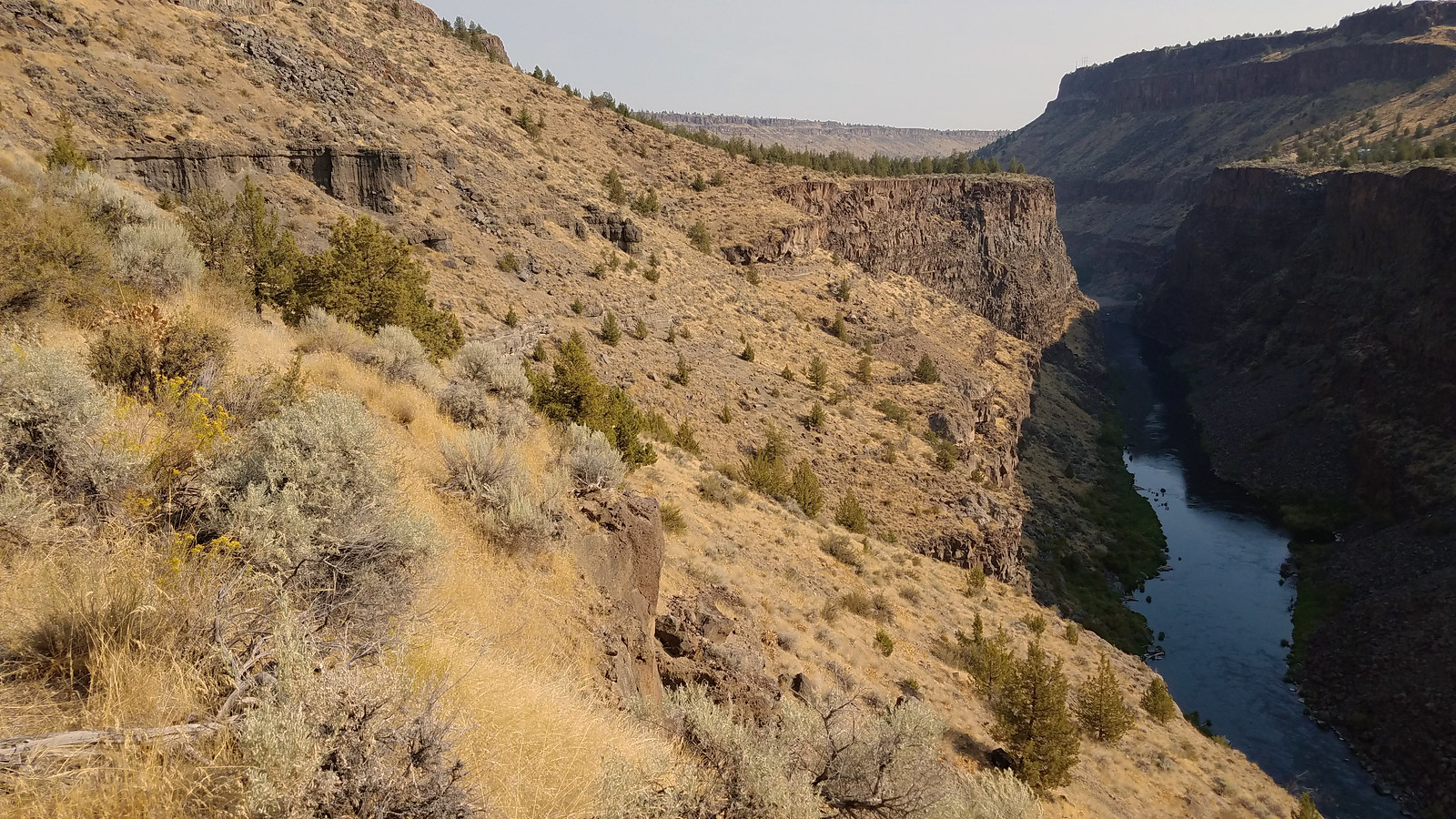This image captures a dramatic canyon landscape with a river running through its depths. The canyon walls are steep and towering, with rocky outcroppings that plunge straight down. The river, appearing blue and shaded, winds from the bottom right and stretches toward the center of the image, adding a dynamic element. The terrain is predominantly tan and brown, characterized by sparse vegetation. There are scattered shrubs and grasses, which vary in color from light green to pale yellow and sage, contributing to the arid and starkly beautiful atmosphere. The ground features numerous small cliffs and protrusions, indicative of a rugged and dry environment where vegetation is sparse and primarily consists of dead grass. The sky above is clear and cloudless, suggesting it's either early morning or mid-afternoon, casting natural light over this majestic, yet desolate, scenery.